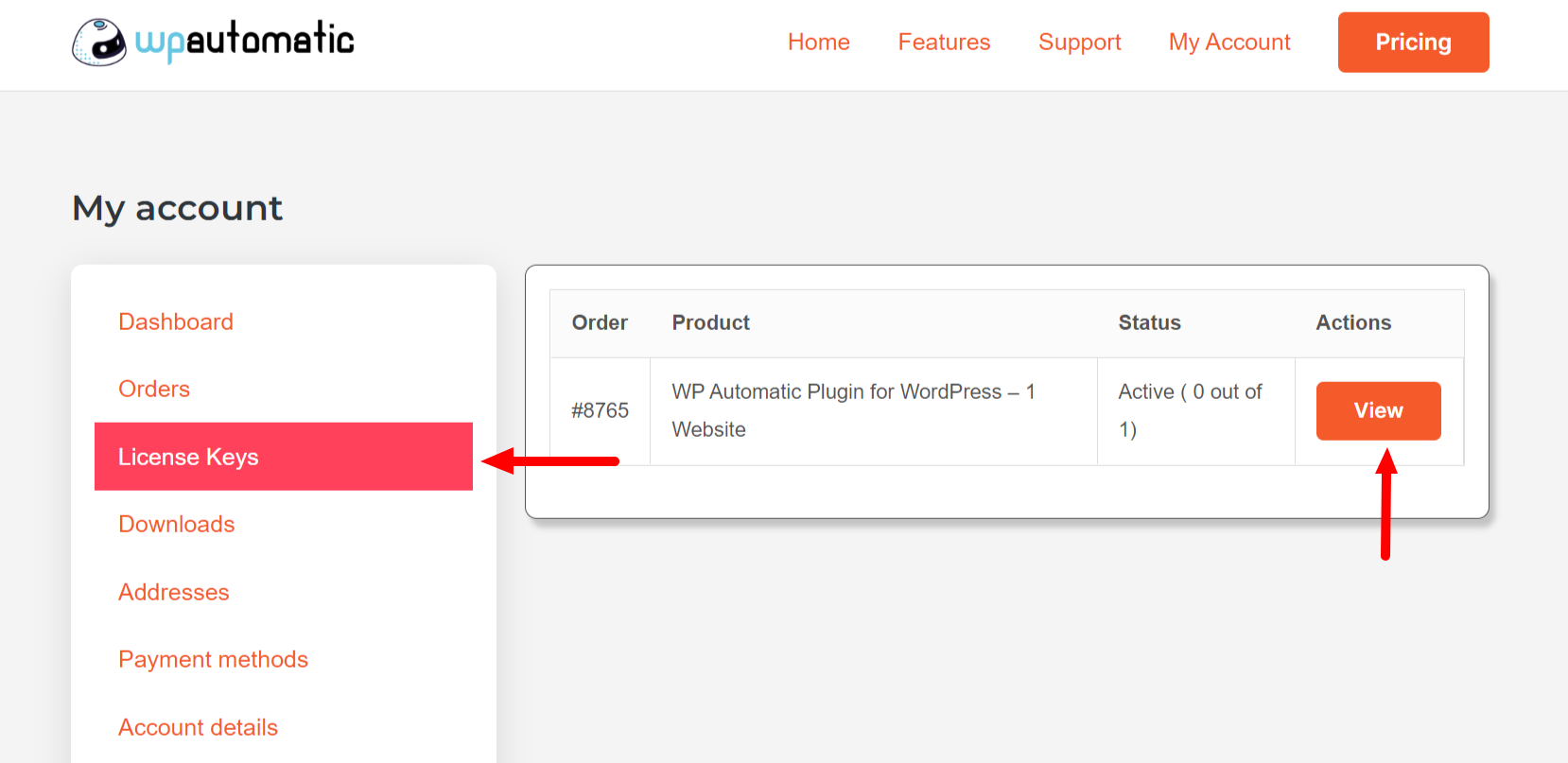This image shows the "WP Automatic" web page on the "License Key" section. In the upper left corner is the "WP Automatic" logo and name, and in the top right there are tabs for "Home," "Features," "Support," "My Account," and "Pricing." Below this top menu, secondary tabs include "My Account," "Dashboard," "Orders," "License Key" (highlighted), "Downloads," "Addresses," "Payment Methods," and "Account Details."

The primary focus of the page displays information about an order: "Order Number 8765" for the "WP Automatic Plugin for WordPress," licensed for "one website." The status is "active," indicated as "0 out of 1 is active." There is also an action button labeled "Click View," presumably for activating or managing the plugin. This page essentially showcases the administrative side of managing a WordPress plugin provided by a third-party vendor, "WP Automatic," which specializes in creating and selling such plugins for the WordPress platform.